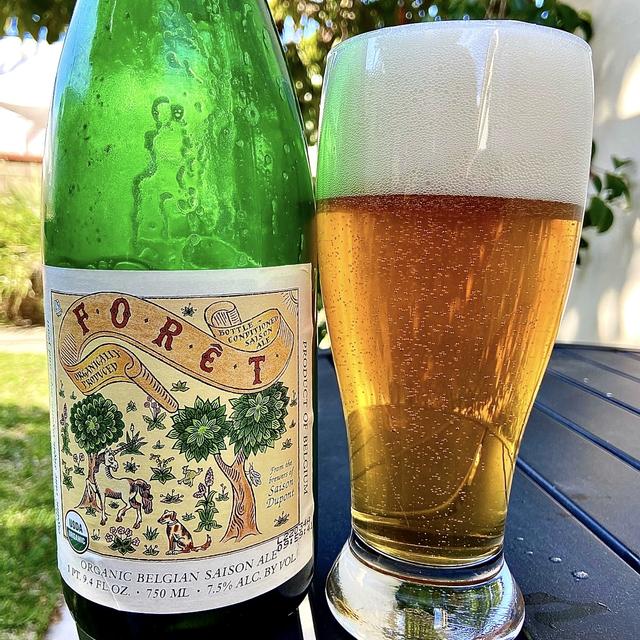A detailed close-up image of a bottle of beer and a glass filled with beer, both placed on a dark wooden table. The bottle is a green, opaque glass with a white label featuring red letters spelling "Foret". The label, resembling old-style parchment, showcases an intricate drawing of two trees, several bushes, a small dog, and a white horse standing on yellow sandy ground. Below this, the label declares it as an organic Belgian ale, with specifics including "one pint 9.4 fluid ounces", "50 milliliters", and "7.5% alcohol by volume".

Next to the bottle, a clear glass goblet holds the beer, with approximately two-thirds liquid and one-third thick white foam crowning the top. The beer itself is golden and effervescent with tiny bubbles rising through it.

Both the bottle and the glass are positioned on a black outdoor table, against a backdrop featuring a white wall, a tree, some grass, and a line of bushes marking the edge of a backyard.